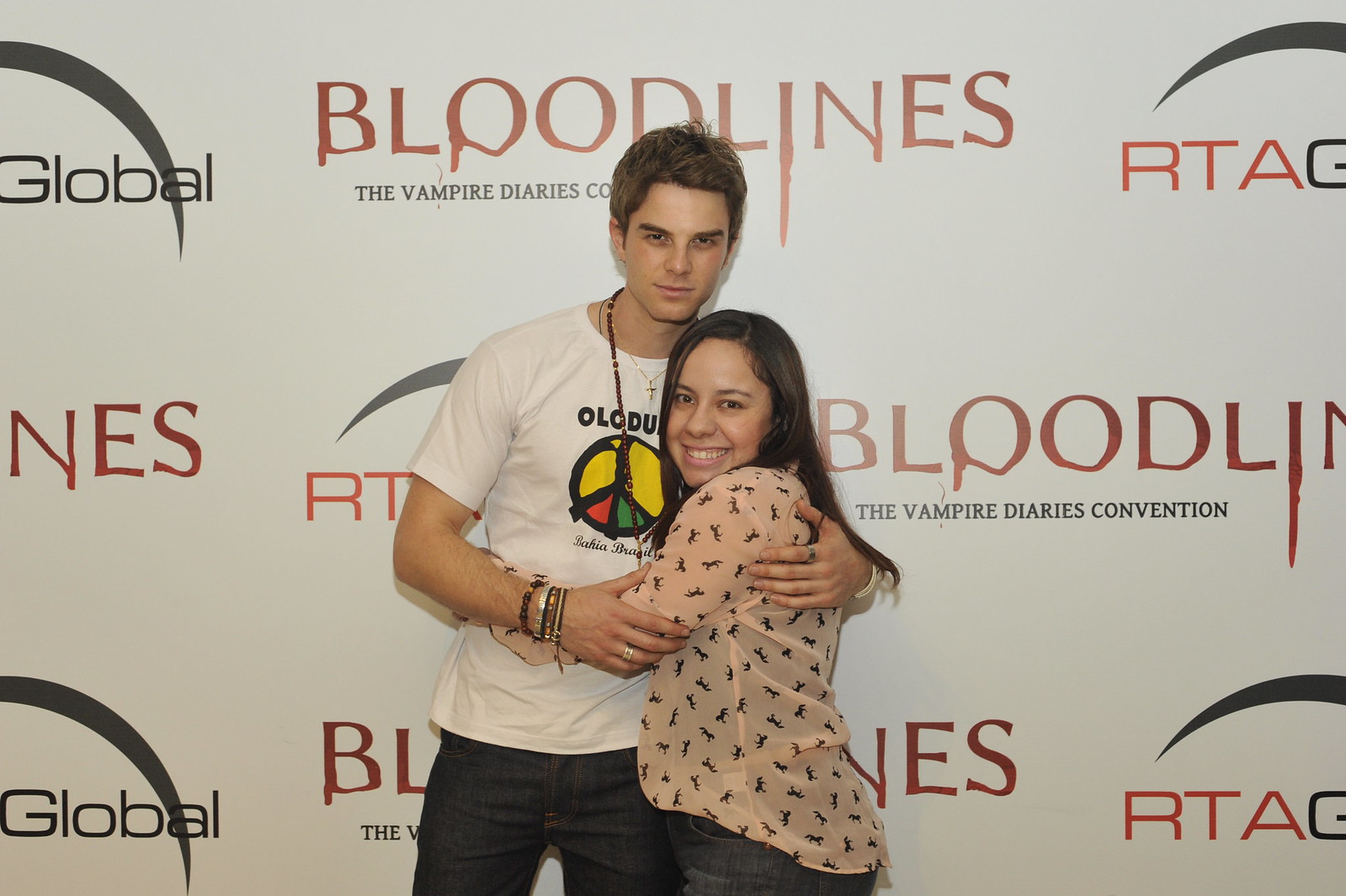A young man and a young woman are warmly embracing in front of a promotional banner for "The Vampire Diaries" convention, which prominently displays the phrases "Bloodlines: The Vampire Diaries Collection" and "RTA Global" with a black arch. The man, who has slightly poofy brown hair, is wearing a white short-sleeved shirt featuring a peace symbol in the center and is adorned with numerous bracelets and rings. He is tilting slightly to the right, wrapping his arms around the young woman. The woman's long black hair cascades down below her shoulder blades. She is dressed in a light pink long-sleeved shirt decorated with small black spider motifs and has her face turned back towards the camera, smiling. Both are wearing black pants, and behind them, the wall is a light gray color, creating a subtle backdrop to their affectionate pose. This appears to be a meet-and-greet event, likely capturing a moment between a fan and a star of the show.